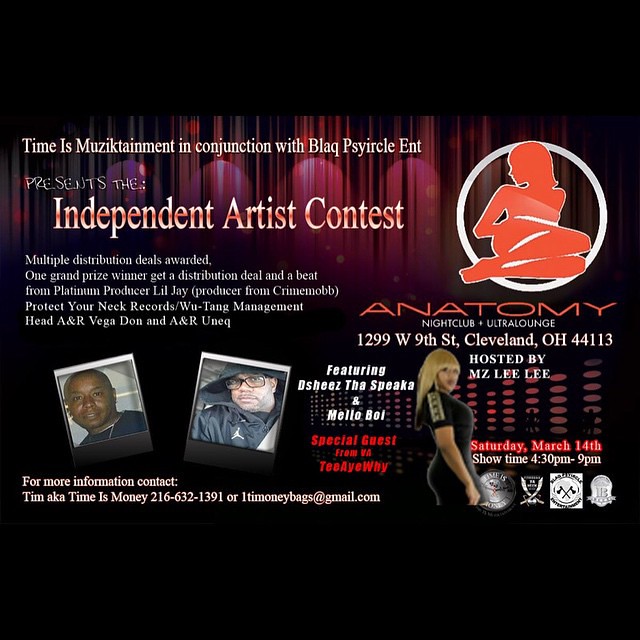An advertisement for an independent artist contest hosted by Time is Music Entertainment in conjunction with Black Physical E&T and held at the Anatomy Nightclub Ultra Lounge, located at 1299 West 9th Street, Cleveland, Ohio, 44113. The event takes place on Saturday, March 14, with showtime from 4:30 PM to 9:00 PM, and is hosted by Mz Lily.

The top-left corner features white text, announcing "Time is Music presents the Independent Artist Contest," with the promise of multiple distribution deals being awarded. The grand prize winner will receive both a distribution deal and a beat from platinum producer Lil J, as well as accolades from Protect Ya Neck Records/Wu-Tang Management head A&R Vegadon and A&R UNEQ.

Two headshots are featured underneath the text: one of a bald African-American man wearing a blue shirt and chain, and another of a white man in glasses and a black hoodie. Next to these photos, it lists the featured artists Ojez Da Speaks and Emilio Pohl. Additionally, a special guest from VA, named Tec YY, is mentioned.

To the right, there is a silhouette of a woman in a sleek black dress with a light green stripe over her shoulder, her blonde hair slightly covering her bangs. Above her is an orange silhouette of a woman laying on her side, with artistic white streaks decorating her form.

At the bottom of the poster, contact details are provided for further information: Tim, aka TimeisMoney, can be reached at 216-632-1391 or via email at onetime1moneybags@gmail.com. The design is punctuated with four decals of varying colors, adding visual interest to the black background.